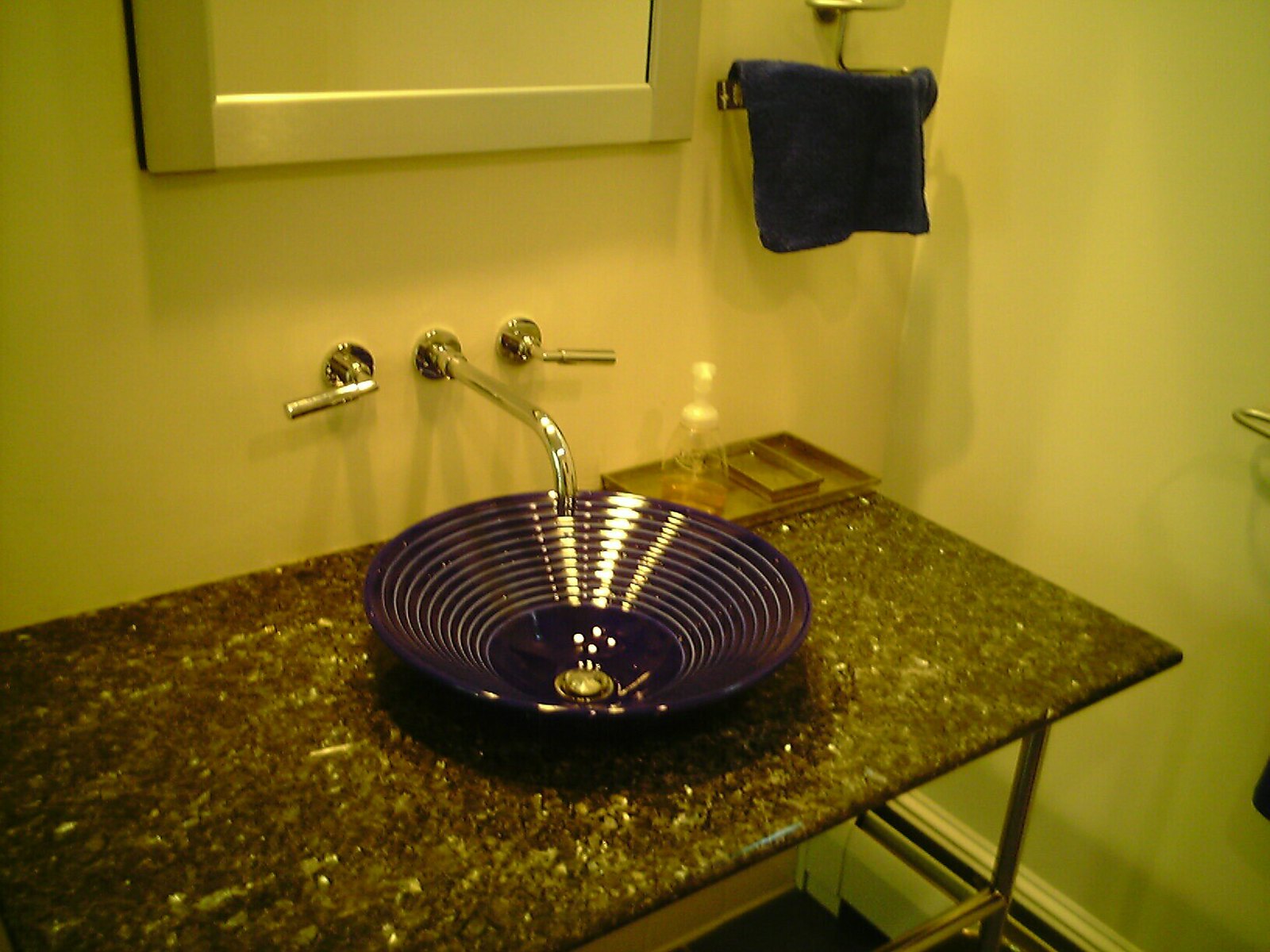The image showcases a modern bathroom sink with a minimalist design. The sink features a sleek, thin countertop and a wall-mounted faucet. The faucet extends out from the wall and curves downward, directing water into a black bowl-shaped basin. This basin is adorned with concentric rings and has a golden drain at its base. Flanking the faucet are two wall-mounted handles that control the water flow. Above the faucet, a mirror with a white border adds to the contemporary aesthetic. On the right side of the setup, a purple towel hangs on a wall-mounted towel holder. Additionally, a small dish on the countertop holds a plastic soap container, adding a practical touch to the elegant setting.